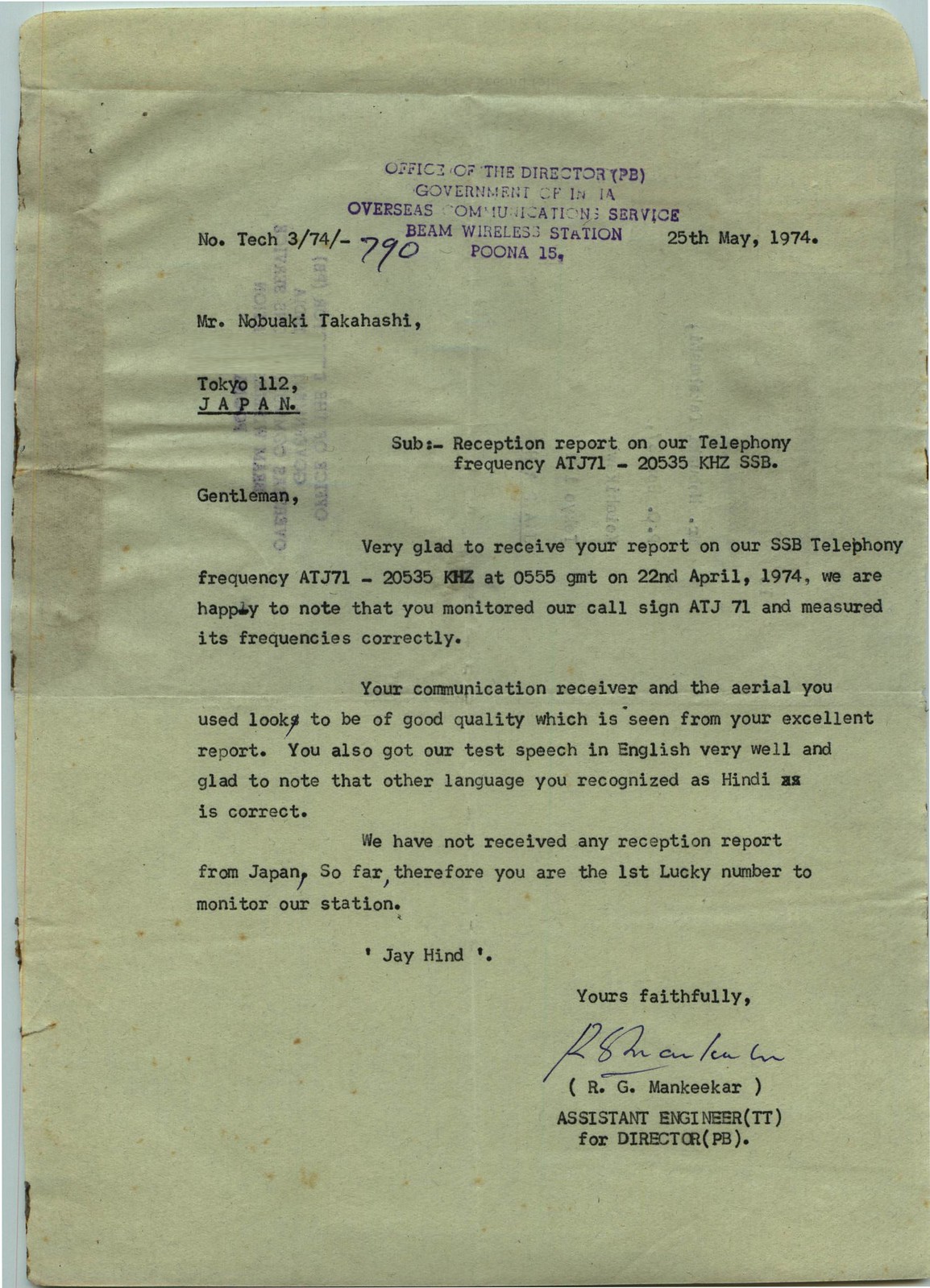This image features an aged, typewritten letter stamped at the top in purple ink with the header: "Office of the Director, PB, Government of Overseas Communication Service, Beam Wireless Station, Puna 15." To the right of the header is the date, "25th May 1974," and to the left is a reference number, "TAC 374-790." The letter is addressed to Mr. Nobuaki Takahashi in Tokyo 112, Japan. It acknowledges the receipt of a report on their SSB telephony frequency, ATJ 71-20535 KHz, and expresses gratitude for monitoring the call sign, ATJ7L, and its correct frequency measurement. The letter, which appears to have been folded in the middle, is signed at the bottom with "J Jai Hind Yours faithfully," and "R.G. Mankeer, Assistant Engineer IT for Director," followed by "PS" in parentheses.